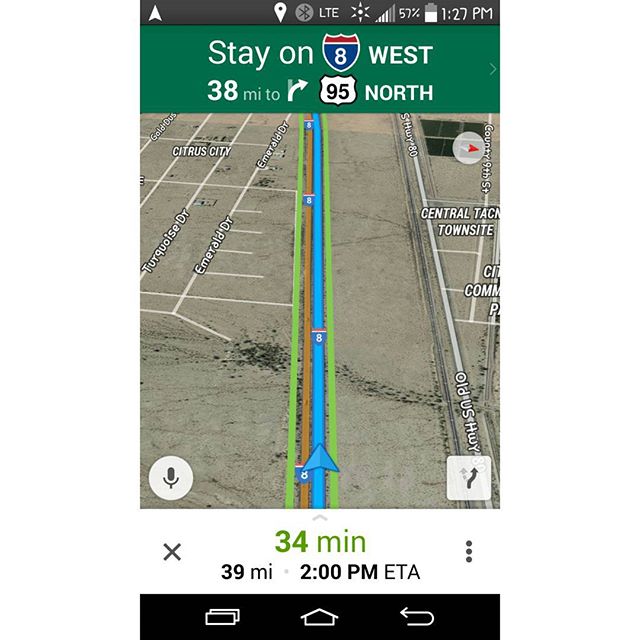This is a mobile device screenshot showing a Google Maps-like navigation screen. Dominating the center is a map with bright blue lines indicating the primary route, alongside side streets and a major highway. At the top, a green banner instructs the user to "Stay on Highway 8 West, 38 miles to turn on 95 North," and includes a right-turn arrow. The top section also features standard mobile icons: Bluetooth, LTE connection, a 57% battery charge, and the current time, 1:27 PM. Street names are displayed alongside the route, with additional colors like green and orange indicating various road conditions. At the bottom, details such as an estimated travel time of 34 minutes, a distance of 39 miles, and an estimated time of arrival at 2:00 PM are given. Below this information, there are icons including a microphone inside a white circle, a detour symbol inside a white square, a white rectangle with an "X," and three vertical black dots on the far right. Various mobile buttons, such as the back and home buttons, are also visible.